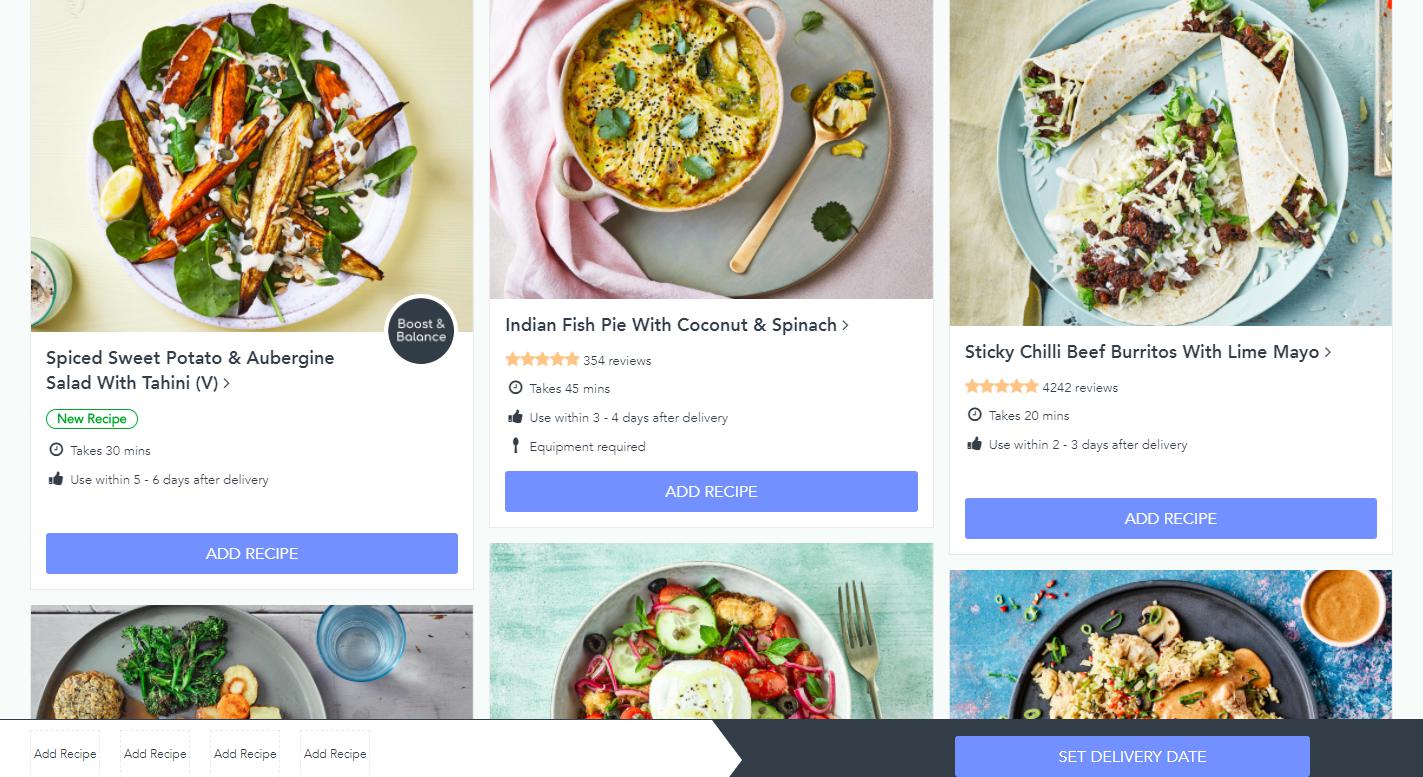This screenshot is from a culinary site that offers both recipe guidance and meal delivery options. The screenshot features six professionally photographed dishes displayed in a top-down view, with accompanying text describing the meals. Only the text for the top three dishes is fully visible, while the bottom three are partially cut off, still showcasing enticing images.

1. **Spiced Sweet Potato and Aubergine Salad with Tahini**:
   - **Description**: A new recipe featuring a vibrant spiced sweet potato and aubergine salad drizzled with creamy tahini.
   - **Preparation Time**: 30 minutes.
   - **Usage**: Best if consumed within 5-6 days after delivery.
   - **Action**: Light purple button labeled "Add Recipe."

2. **Indian Fish Pie with Coconut and Spinach**:
   - **Description**: An exotic Indian fish pie infused with rich coconut flavors and fresh spinach.
   - **Rating**: 5 stars based on 354 reviews.
   - **Preparation Time**: 45 minutes.
   - **Usage**: Best if consumed within 3-4 days after delivery.
   - **Required Equipment**: Spoon icon indicates some required utensils.
   - **Action**: Light purple button labeled "Add Recipe."

3. **Sticky Chili Beef Burritos with Lime Mayo**:
   - **Description**: Spicy and flavorful sticky chili beef burritos complemented by zesty lime mayo.
   - **Rating**: 5 stars based on 4,242 reviews.
   - **Preparation Time**: 20 minutes.
   - **Usage**: Best if consumed within 2-3 days after delivery.
   - **Action**: Light purple button labeled "Add Recipe."

While partial text can be seen below the three main dishes, the visible images hint at diverse dishes including a possible spinach and cucumber salad and a chicken dish. All dishes feature an "Add Recipe" button, suggesting the ease of adding these items to a cart or meal plan.

Lastly, a light purple button on the right side of the screenshot is labeled "Set Delivery Date," indicating functionality for scheduling meal deliveries.